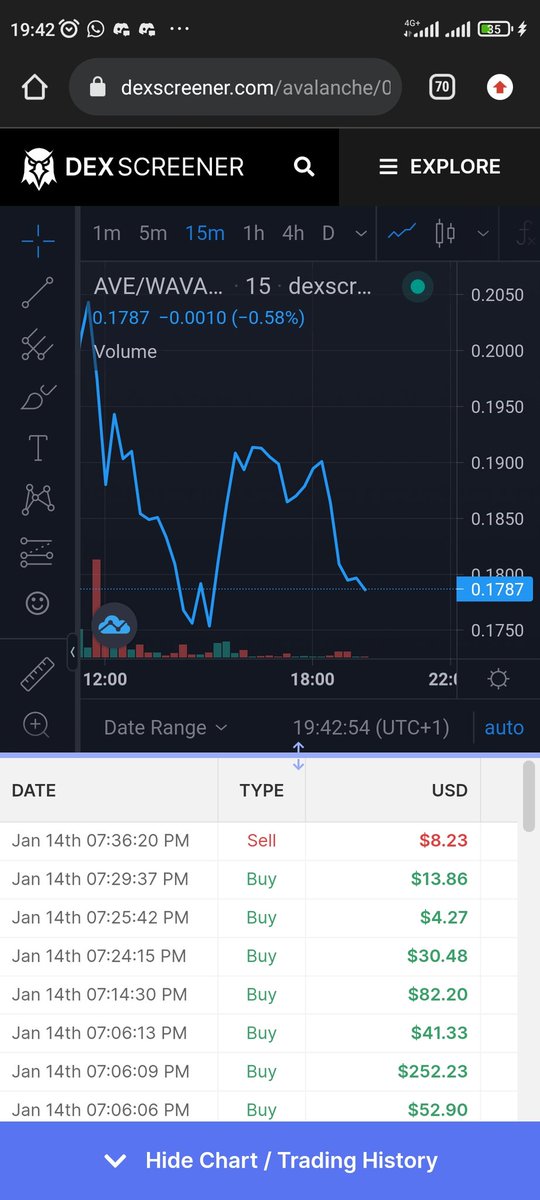The image displays a screenshot of a mobile phone screen, predominantly black in the background. At the top of the screen, there's a URL partially visible: "dexscreener.com/avalanche/...". Just beneath the URL, an icon of an eagle’s face accompanies the text.

Centrally positioned within the image is a line graph, colored blue. The graph starts at a high point, then sharply descends, slightly rises, and again drops drastically. Below the line graph, a corresponding bar graph shows similar high and low fluctuations in volume.

At the bottom of the image, different timestamps are noted, all pinpointing to January 14th, such as 7:36 PM. Transactions are detailed below the graphs, indicating that an item was sold for $8.23 (highlighted in red), whereas the buying transactions are marked in green.